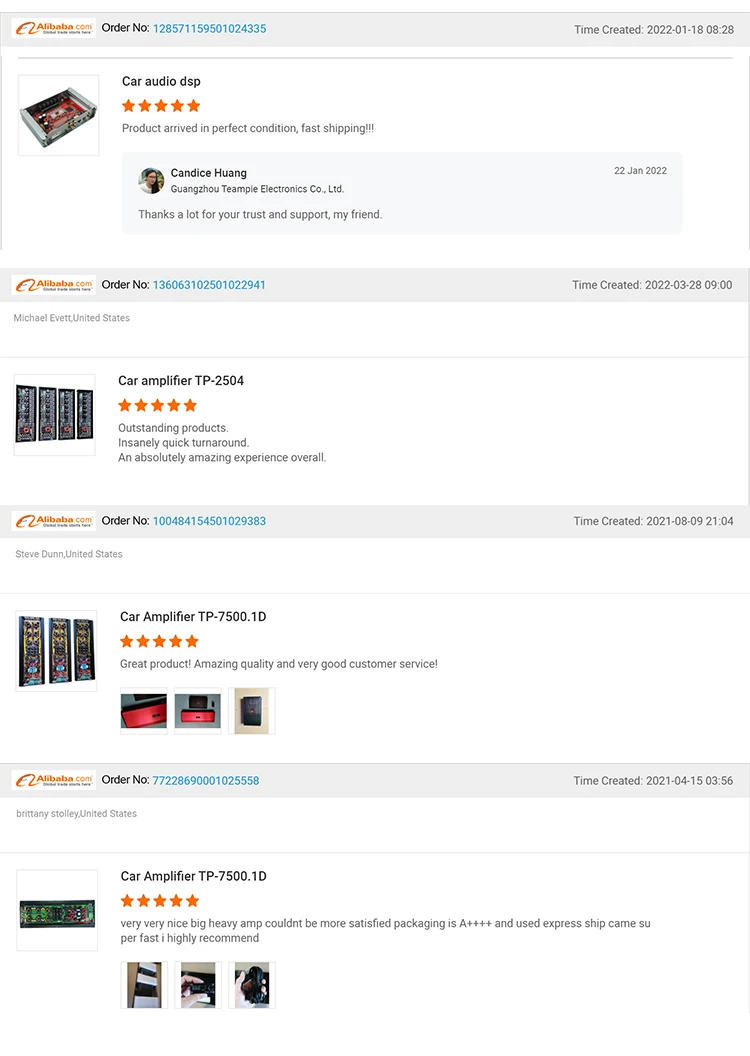This image from Alibaba.com displays a collection of various car parts available for purchase, along with detailed order information and customer feedback, showcasing high levels of satisfaction.

At the top of the image, the Alibaba.com logo is prominently displayed alongside the order number 128-571-1159501024. The created timestamp reads 2022-01-18 08:28. Below this, the product description "Car Audio DSP" is followed by a note stating the product arrived in perfect condition, with fast shipping. The item has received a 5-star rating. The image to the left depicts a metal box with several red and black components. The customer, Candace Hwang from Gaozhong Teampool Electronics Co. LTD, expresses gratitude for the support, showcasing a profile picture and a date of 2022-02-02.

The next order listed is number 136-063-102-501022941, with a creation time of 2022-03-28 at 09:00. This order pertains to a car amplifier model TP-2504, shown in the picture to the left, and has garnered a 5-star rating. The feedback highlights outstanding products, an insanely quick turnaround, and an overall amazing experience. The customer, Michael Everett, is based in the United States.

Following this, order number 100484154501029383 has a timestamp of 2021-08-09 at 21:04 military time. The user, Steve Dunn from the United States, ordered a car amplifier model TP-7500.1D. This product also has a 5-star rating and praise for its great quality and excellent customer service, accompanied by three product images at the bottom and a picture to the left.

The final order detailed in the image is number 7722866900010225558, created on 2021-04-15 at 03:56. The customer, Brittany Stolle from the United States, ordered another car amplifier model TP-7500.1D. The product received a 5-star rating with a review highlighting it as a very nice, big, and heavy amp with excellent packaging and express shipping. The feedback concludes with a high recommendation, accompanied by three pictures below and an additional image to the left.